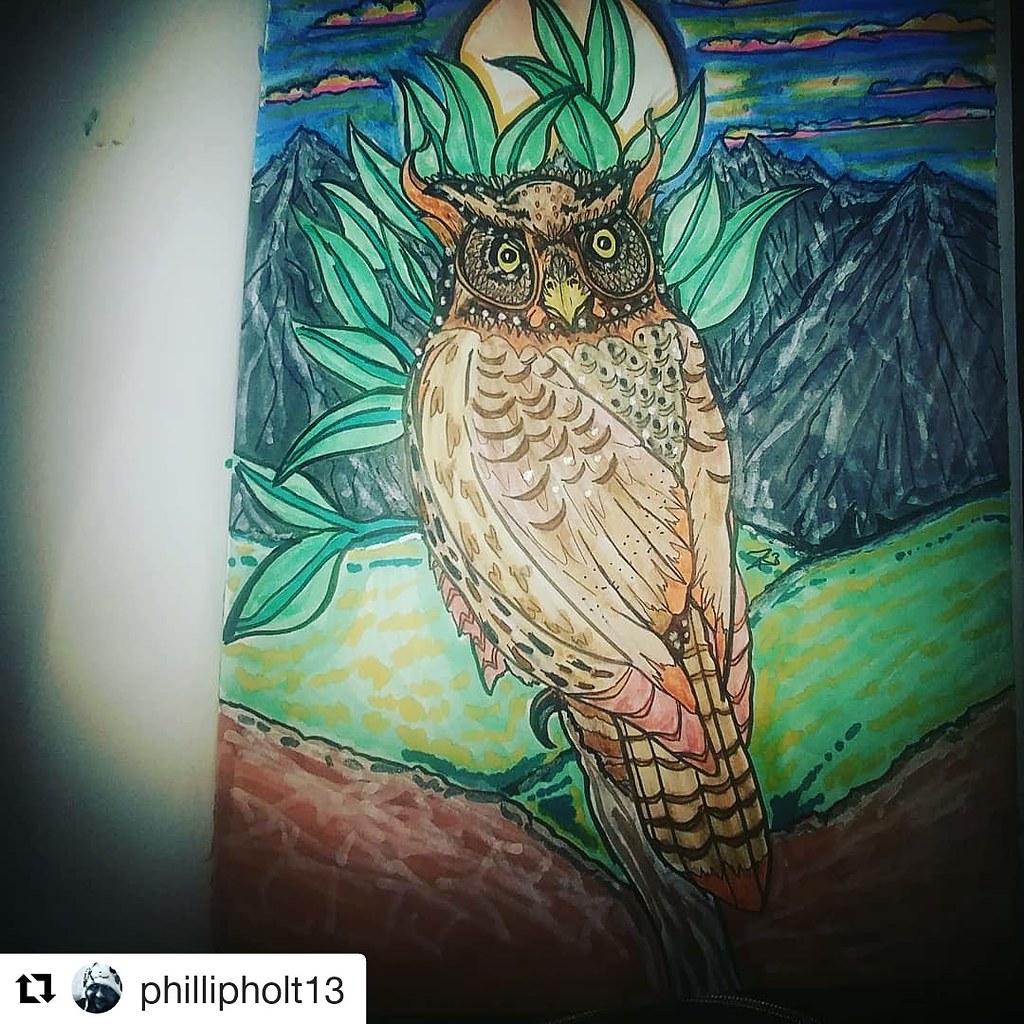This is a square-format, color photograph showcasing a vibrant, intricate drawing of an owl. The owl sits on a green and brown stem, its body facing away but its head turned to stare directly at the viewer with its wide, yellow eyes and stern, serious expression. The owl's feathers are a rich mix of browns, blacks, and yellows, with touches of red on its wings and a distinctive yellow beak framed by black markings. Surrounding the owl, a backdrop of lush greenery, distant mountains, and a blue, cloudy sky with a full moon create a picturesque scene. The entire drawing rests on a white table, illuminated by a light source from the left, and in the lower left corner, there is a square arrow emblem, a small black-and-white photo of a man's face, and the name "Philip Holt 13."